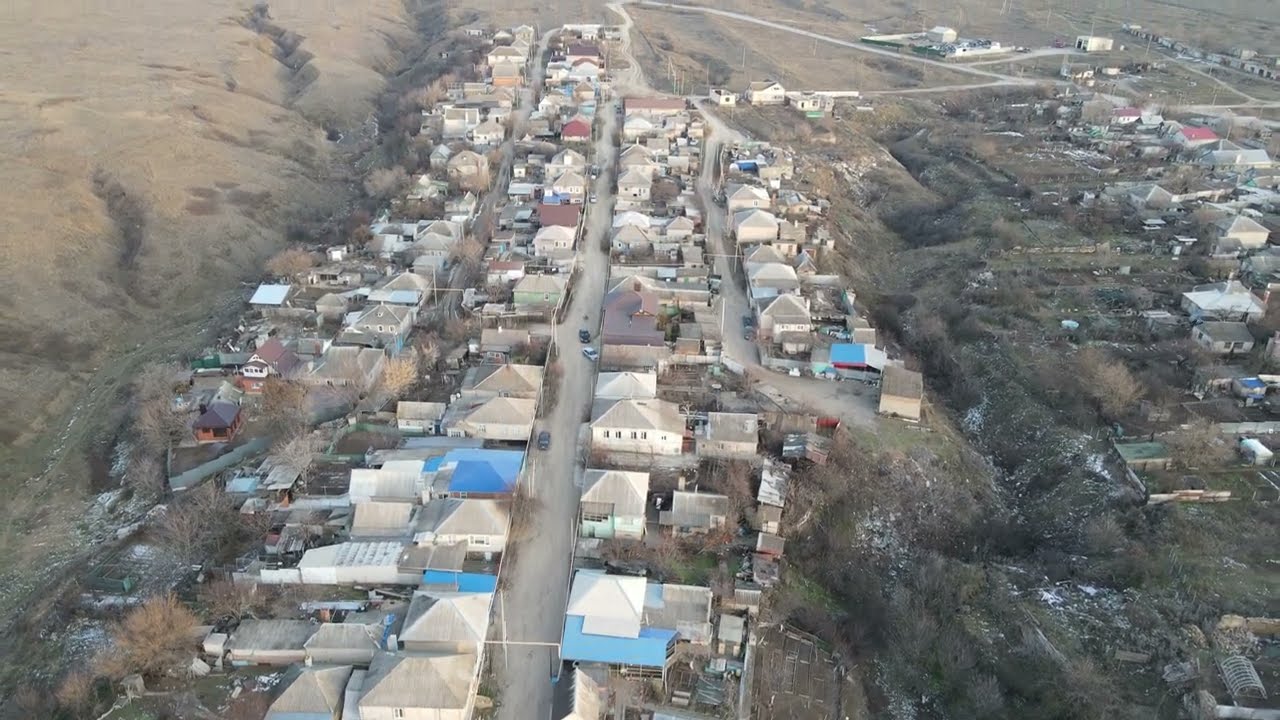This aerial color photograph captures a rural neighborhood situated on a hilly, somewhat rugged terrain. A main road runs vertically through the center of the image, flanked by clusters of buildings, likely houses, with a mix of blue, gray, and brown roofs. The neighborhood looks somewhat crowded and is possibly aging, with structures estimated to be around 30 to 40 years old. The landscape features a hill rising on the left side, leading up to more houses, and descending on the right toward a valley with additional buildings and trees. The colors appear dull and washed out, suggesting poor photographic quality. The area seems to lack meticulous upkeep and is far from metropolitan, with approximately 50 to 100 houses visible in total. Several smaller roads branch off from the main road, intersecting with the rows of houses, highlighting the layout's complexity within this non-urban setting.